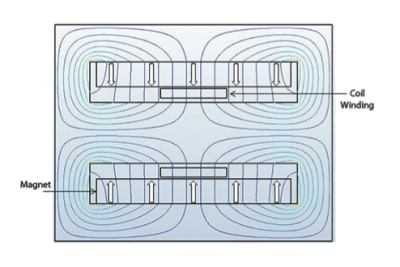This detailed illustration provides a scientific explanation of magnets and coils. The central focus is a square-like rectangular dark blue box with a light blue interior. Inside, there are four light blue, vaguely circular shapes, arranged two on the top and two on the bottom, each with swirling purplish patterns. Resting above these shapes is a long rectangular box divided into distinct sections, where some sections feature arrows pointing downward. A similar rectangular box is positioned at the bottom of the image, with arrows pointing upward. The word "MAGNET" with an arrow leading into the rectangular area is located at the bottom, while "COIL WINDING" with an arrow pointing to the upper rectangle is found on the right-hand side. The overall background of the image is light blue, and the entire diagram is set against a white background.